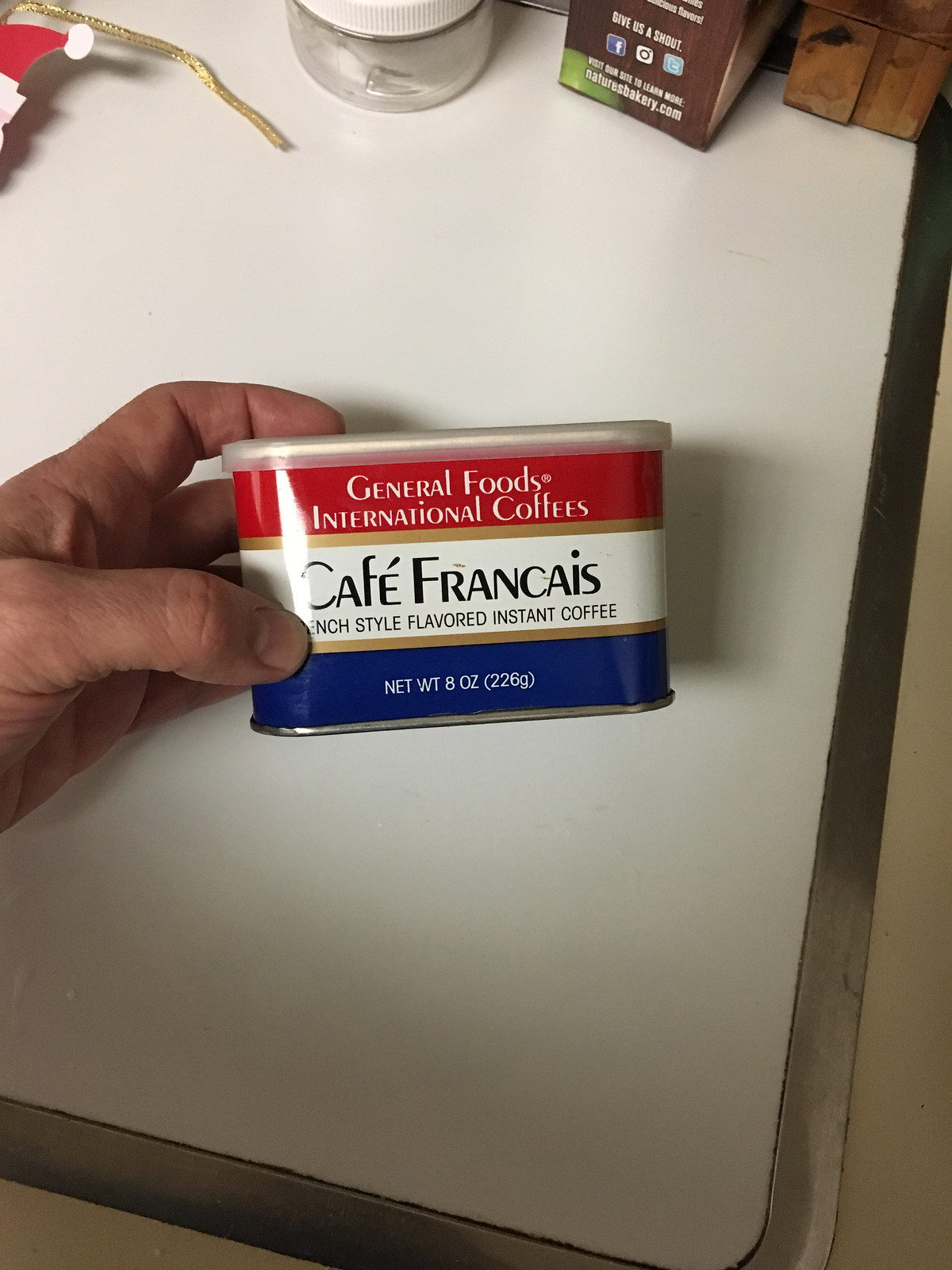The photograph captures a person's left hand with short, unpainted nails, holding a tin of General Foods International Coffees Café Francais, French-style flavored instant coffee. The tin, decorated in the colors of the French flag—red at the top, white in the middle, and blue at the bottom, each section separated by a thin gold band—features a clear plastic lid. The label at the top reads “General Foods International Coffees” in white text on the red band, followed by “Café Francais French-Styled Flavored Instant Coffee” in black on the white band. The blue band at the bottom states the net weight of 8 ounces (226 grams). The hand tilts the can towards the camera, revealing these details against a somewhat dated, white kitchen countertop with a silver metal border. In the background, light filters in from the top left corner, providing minimal illumination. Along the top of the image, a festive Christmas gift tag featuring a Santa hat dangles, and nearby are a glass jar with a white plastic lid, a box of baking goods, and possibly the base of a wooden knife holder. The overall scene combines holiday decor with a nostalgic touch of the kitchen setting.